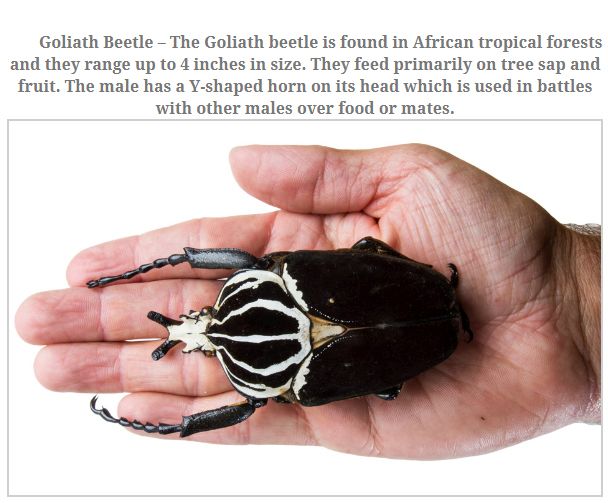In the image, a man holds a sizable Goliath beetle in his right hand, with the beetle's body extending from the tip of his index finger to about an inch away from his wrist. The beetle is predominantly black, featuring distinctive white stripes on its head and a beige section above its wings, which are tipped with white. The insect, about as wide as three fingers, boasts thick antennae and two long arms. Above the photo, a paragraph in gray text on a white background provides detailed information about the beetle: it is found in African tropical forests, can grow up to four inches in size, and primarily feeds on tree sap and fruit. Male Goliath beetles are noted for their Y-shaped horns, which they use in battles over food or mates.